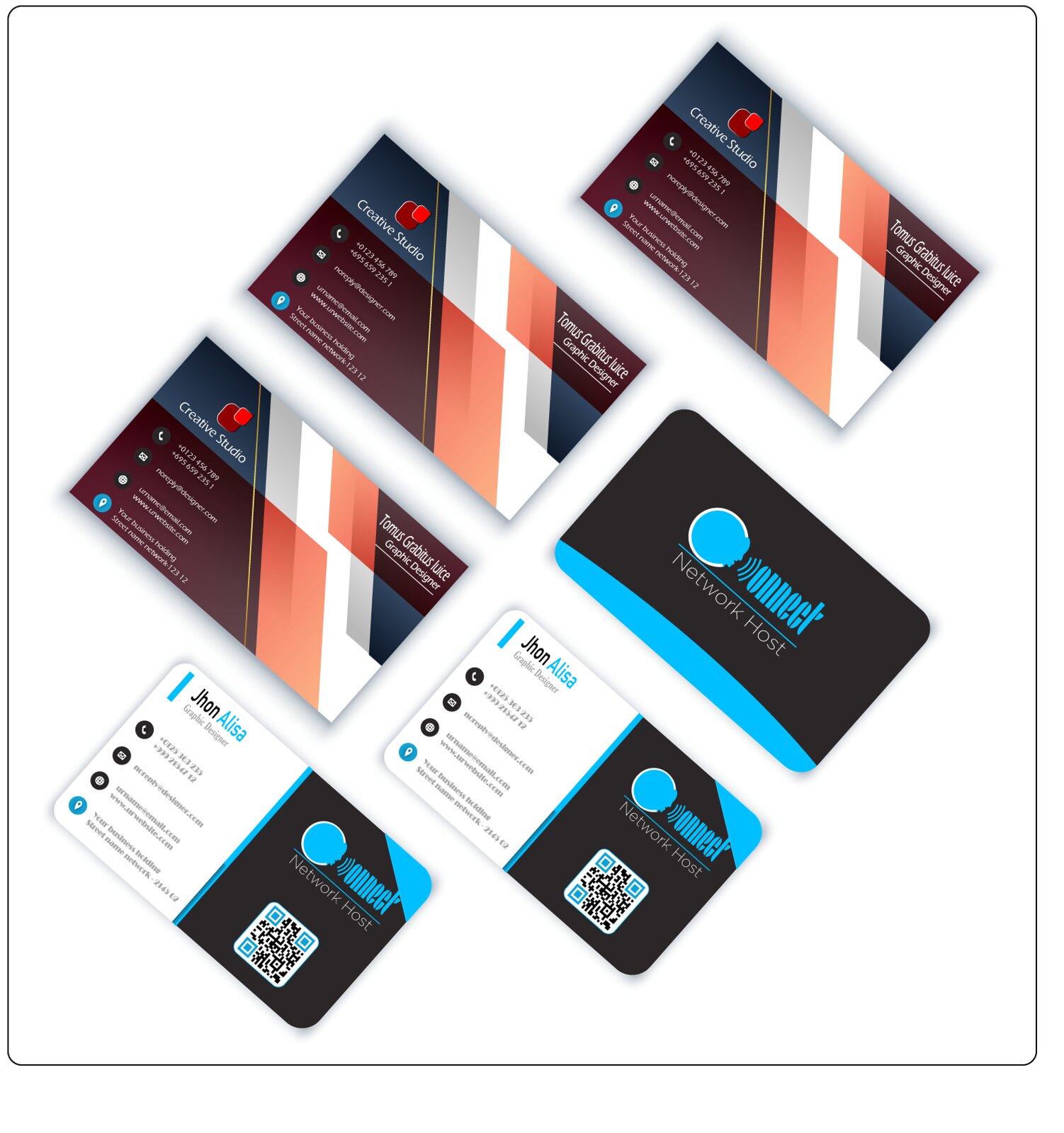The image showcases six business cards arranged in two sets of three. One set belongs to 'Connect Network Host' and features a sleek black background with an eye-catching curved blue line. The front side of these cards prominently displays "CONNECT" in bold dark blue letters, with "Network Host" in dark gray beneath it. On the back, the card details for Johan Alisa, a graphic designer, are provided in two-tone text, with Johan in black and Alisa in blue. This side also includes a QR code to the right and aligned contact icons for phone, email, web, and GPS, all displayed in white against dark gray or blue circles. 

The second set of cards is for Thomas Grabius Lucy from Creative Studios. These cards exhibit a vibrant design featuring a mix of maroon, red, pink, dark gray, white, and blue trapezoidal shapes. Within these shapes, the card prominently states "Creative Studio" in white text over a golden line. Below, there is a maroon square with creative designer Thomas Grabius Lucy's name, contact details, including phone numbers, email addresses, and a website. The card features graphical symbols for phone, email, web, and GPS against various colored backgrounds. Like the first set, these details are organized next to three business cards' repetitions within the image. Both sets of cards provide comprehensive contact information, showcasing sophisticated, visually distinct designs for their respective services.